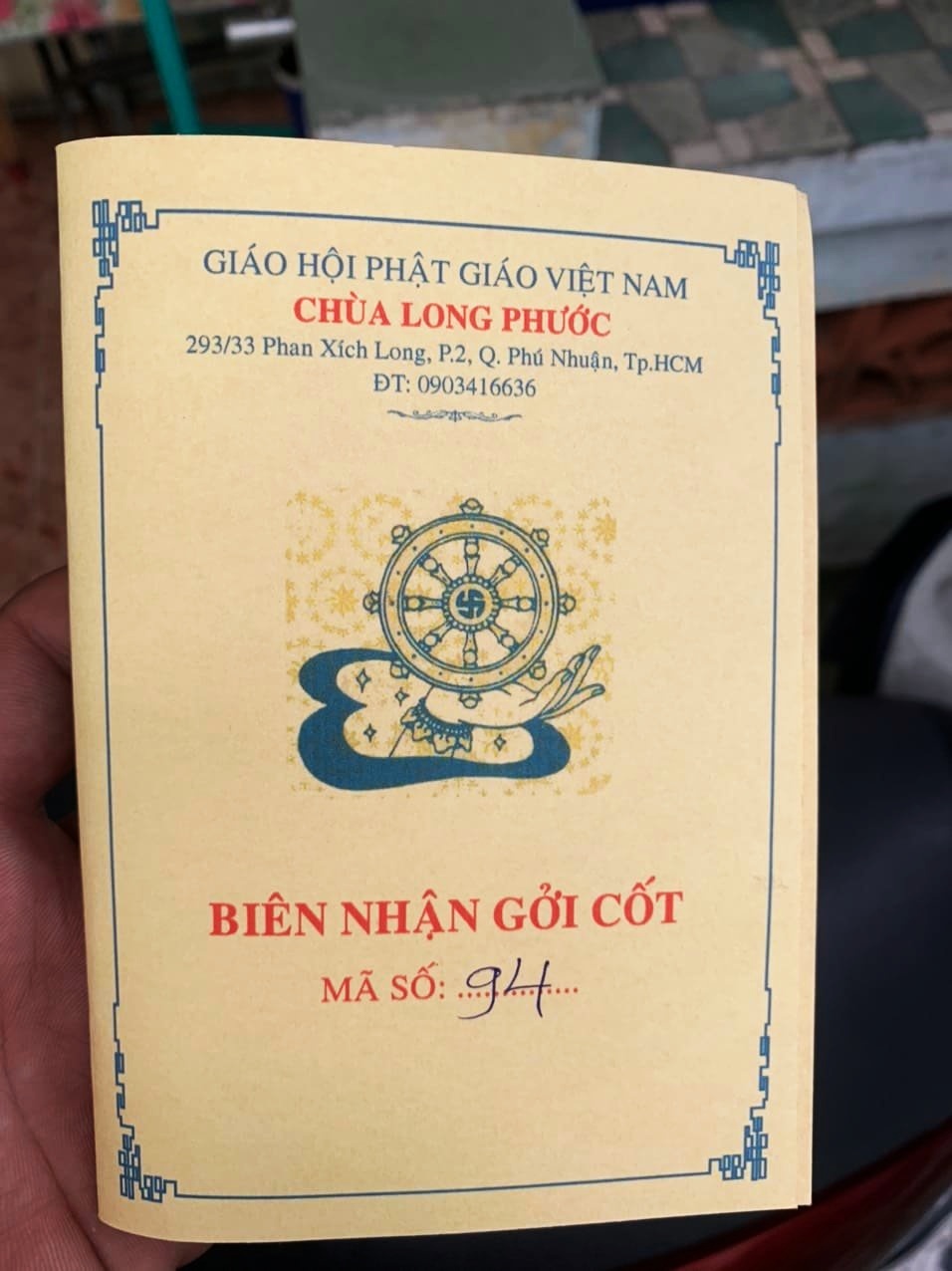This image depicts a standing, folded beige piece of paper, prominently bordered with blue, giving it an elegant and formal appearance. At the top of the paper, there is blue text that reads "Giáo Hội Phật Giáo Việt Nam," suggesting a Vietnamese origin. Below this, bold red capital letters spell out "Chùa Long Phước," followed by an address in smaller blue text: "293-33 Phan Xích Long P2Q Phú Nhuận, T-PHCM," and a contact number "DT: 0903416636" beneath a subtle decorative squiggly line.

Centrally placed on the paper is a detailed drawing of a woman’s hand, palm up, adorned with a frilly blue and tan cuff, which elegantly outlines her wrist. She holds what appears to be a ship’s steering wheel, intricately designed with alternating blue and tan colors. This imagery possibly suggests guidance or direction and is reminiscent of a ship navigating its course.

Below this artistic centerpiece, in large red capital letters, are the words "BIỂN NHÂN GỢI CỐT." Smaller capital letters in a thinner font spell out "MÃ SỐ," followed by a colon, and the handwritten notation "G4," though some initially interpreted it as "94," indicating the individualized nature of the document.

The overall design and detailed elements suggest that the paper might be ceremonial or official in nature, possibly akin to a brochure or a ceremonial pamphlet, emphasizing Vietnamese culture through its text and visuals.